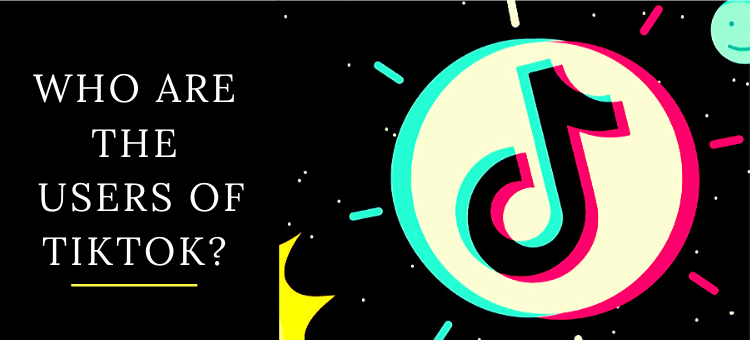This TikTok-themed banner features a black background with a prominent, well-organized design. On the left side, white text reads "Who are the users of TikTok?" with the word "TikTok" underlined by a striking yellow line, adding emphasis. To the right, a large circle stands out with its distinctive dual-tone outline—teal on the left side and hot pink on the right—while its interior is an off-white shade. The center of the circle showcases the TikTok logo, which mirrors the outline's colors: teal on the left and hot pink on the right, set against a black backdrop.

Enhancing the circle’s dynamic appearance, three teal dashes extend outward from its left side like sun rays, joined by a white dash at the top and another at the bottom, and three hot pink dashes on the right side. The background is sprinkled with small white dots, which resemble stars, adding a whimsical touch to the dark canvas. In the upper right corner, a mint green moon with a playful partial smiley face—depicting one eye and a partial grin—adds a charming, celestial element to this engaging and vibrant TikTok banner graphic.